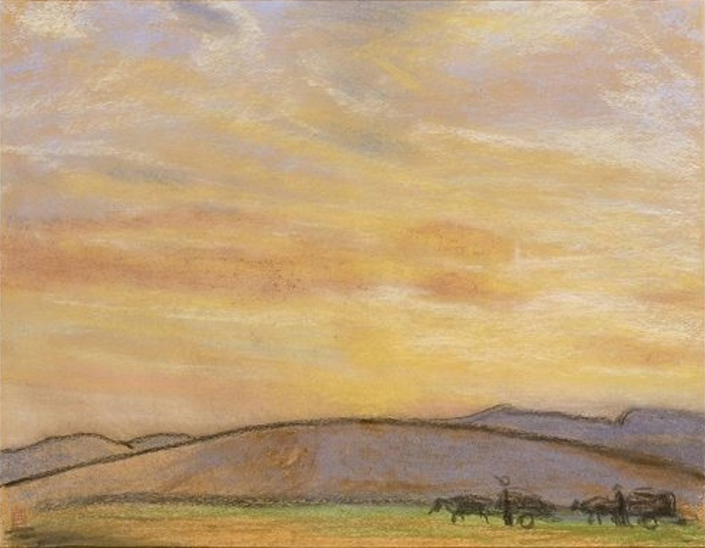The image is a detailed pastel or oil pastel painting featuring a vast and expansive sky that dominates approximately 80% of the composition. The sky exhibits a mesmerizing blend of wispy hues, including shades of yellow, blue, pink, purple, and darker orange. Below the expansive sky stretches a landscape with a low, curved hill or mountain. The foreground showcases green grass, horizontally shaded, with an outlined tan roadway dividing it.

At the bottom, there are small, symbolized figures either journeying with wagons or possibly farmers sowing the soil; the wagons are being pulled by oxen or horses. Among the tiny human forms, one figure seems to be pointing upward. The hilly horizon is marked by less detailed, undulating shapes. On the far left, a mountain peak subtly rises, while to the right, a plateau is visible. The overall scene, though symbolized and lacking intricate detail, captures a scenic, pastoral landscape accentuated by the strikingly vast, dreamlike sky.